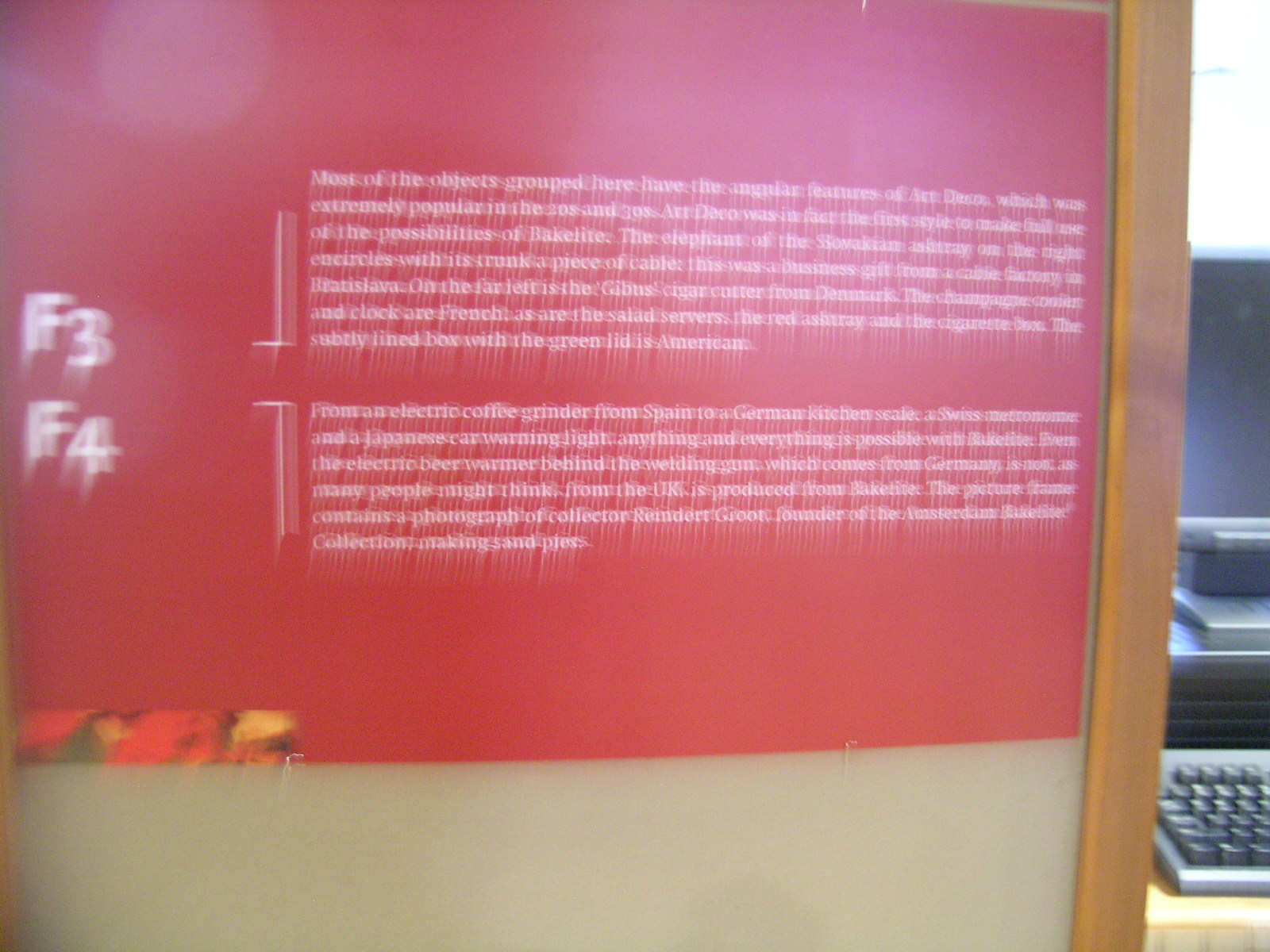The image depicts a very zoomed-in view of a red informational sign with illegible white text due to blurriness. The sign is framed in a light blonde wooden frame that does not fit the full length of the piece of paper, leaving a gap at the bottom filled with a light gray material, possibly the cardboard backing of the frame. The red paper has small white writing, including two paragraphs of text—one at the top left with a small horizontal line followed by a vertical line going up, and another at the bottom left with a similar small horizontal line but with a line going down. Next to the left side of the text, there are labels "F3" and "F4." Additionally, a floral pattern in shades of yellow, orange, and red can be seen at the bottom left. To the right of this image, there is a partial view of a computer setup—a bit of a keyboard with black keys and a silver frame, and above that, a black monitor with a silver trim, with some light reflecting on it.